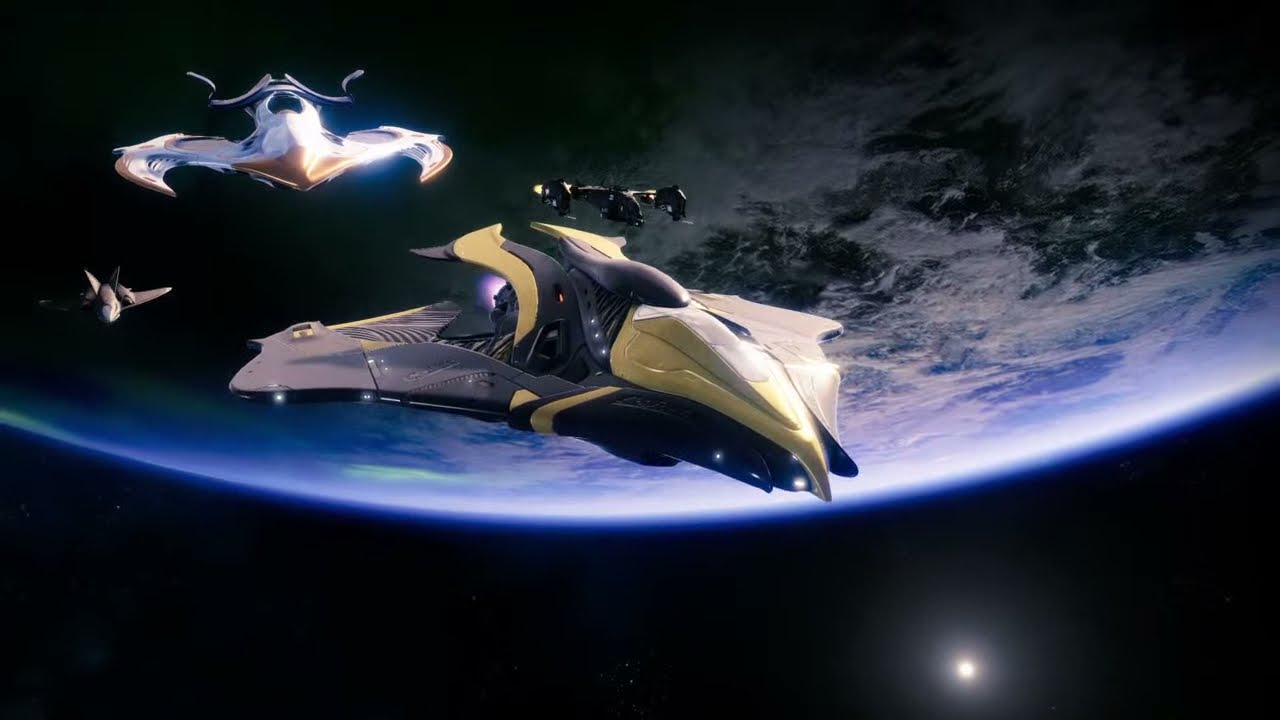The digitally created space scene features the bottom view of a planet, possibly Earth, with a captivating purple glow against the dark black expanse of space. The planet occupies the upper portion of the image, with the top shrouded in darkness and the bottom illuminated by a distant sun positioned in the lower right-hand corner. This sun casts a faint glow, highlighting a single small, glowing dot in the vicinity. Central to the image are four futuristic spaceships of varying sizes and colors. The foremost spaceship is medium-sized and white, followed by a smaller beige or brown craft and a prominently featured gold and black spaceship. Another vessel is situated in the background. This richly detailed graphical or painted scene emphasizes the vivid contrast between the illuminated planet and the stark void of space, creating a striking visual narrative of an interstellar journey.